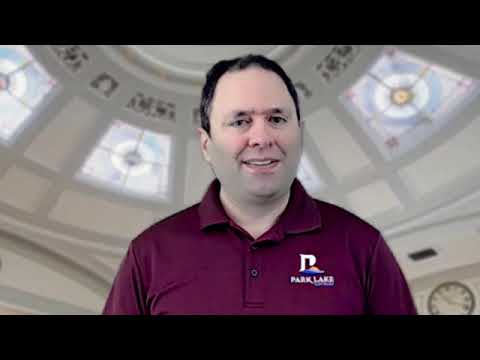The image captures a man in what appears to be a still from a video, likely a promotional or instructional Zoom video. The man, a European-looking individual in his 40s or 50s, has fair skin, sparse dark hair, and a five o'clock shadow. He has an oval-shaped face and is wearing a maroon or burgundy polo shirt with two buttons buttoned up. On the left chest area of his shirt, there is a logo that reads "Park Lake" in white, incorporating a stylized letter "P" with a small wave-like symbol nearby.

The background behind the man is a domed ceiling, possibly modeled after a Capitol building or Basilica Church. This dome is adorned with muted-colored stained glass panels, mainly in shades of blue, forming circular patterns. There is also a clock visible in the bottom right corner of the image, indicating the time as around 4:50. The man's image appears to be superimposed onto this background, giving the scene a somewhat artificial or photoshopped appearance. He is looking directly at the camera with a slight tilt of his head to the right, and his expression seems somewhat frozen or stiff, adding to the impression of an AI-generated image.